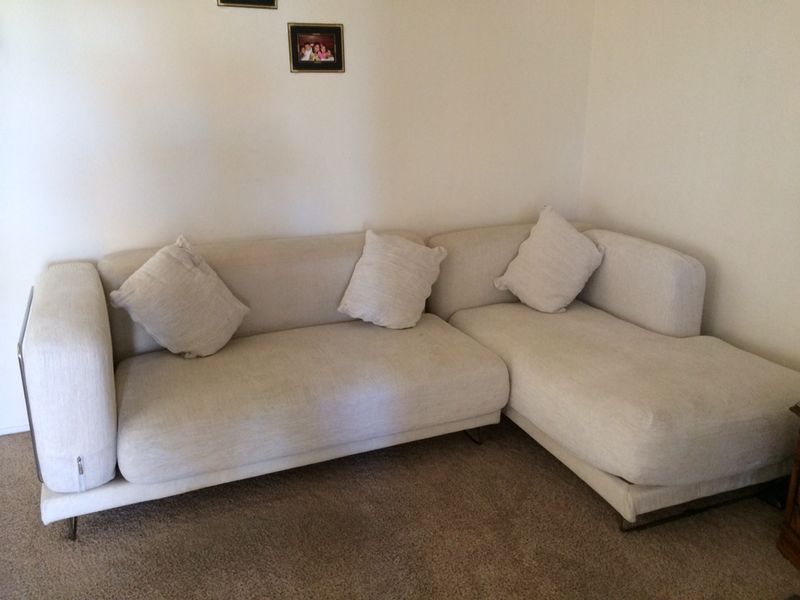The image captures a close-up scene in the corner of a living room where two light beige (off-white) walls converge. Nestled against these walls is a sectional beige couch that wraps around the corner. The couch comprises two distinct parts: one section extends along the left wall and is akin to a chaise lounge, while the other, longer section runs horizontally along the adjacent wall. The overall sectional design suggests a substantial seating area with an armrest on one side and a cohesive backrest.

The floor is covered with a darker beige carpet, enhancing the cozy atmosphere of the room. Additionally, the couch appears to rest on small black legs, which blend seamlessly with the floor. Hanging prominently on the wall above the couch is a framed photograph featuring multiple individuals. To the upper left, the bottom edge of another picture frame is barely visible, hinting at additional wall decor. A small fragment of what looks like a table edge peeks into the frame on the right side, completing the cozy and detailed room setting.